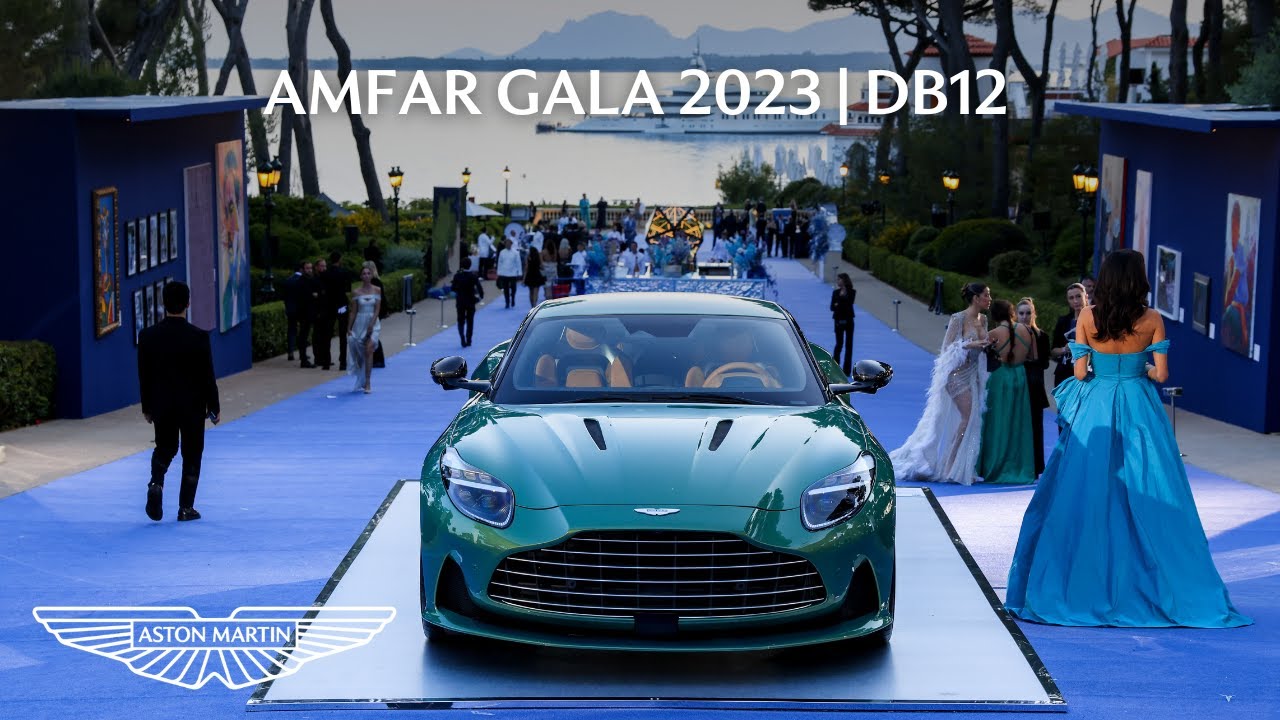The image captures an elegant advertisement for Aston Martin prominently featuring a lustrous green Aston Martin DB12, showcased head-on, revealing its front with shiny brown seats visible through the windshield. The car is perched on a white platform, set upon an extensive deep blue carpet that stretches over a concrete surface, presumably an outdoor venue. To the left and right of this carpeted pathway are two small blue buildings adorned with artwork-like photographs. The scene is part of the Amphar Gala 2023, clearly indicated by the white text at the top of the image.

In the foreground to the right, a woman in a long blue dress with off-the-shoulder straps stands with her back to the viewer, accompanied by other elegantly dressed women, including one in a fluffy white gown and another in a green skirt. Both men and women in exquisite attire can be seen mingling in the background, emphasizing the high-society nature of the event. Behind the gathering, a large white yacht cruises along a nearby waterway, framed by the rolling slopes of distant mountains.

The signature Aston Martin logo, shaped like outspread wings, resides in the bottom left, reinforcing the upscale branding of the advertisement.